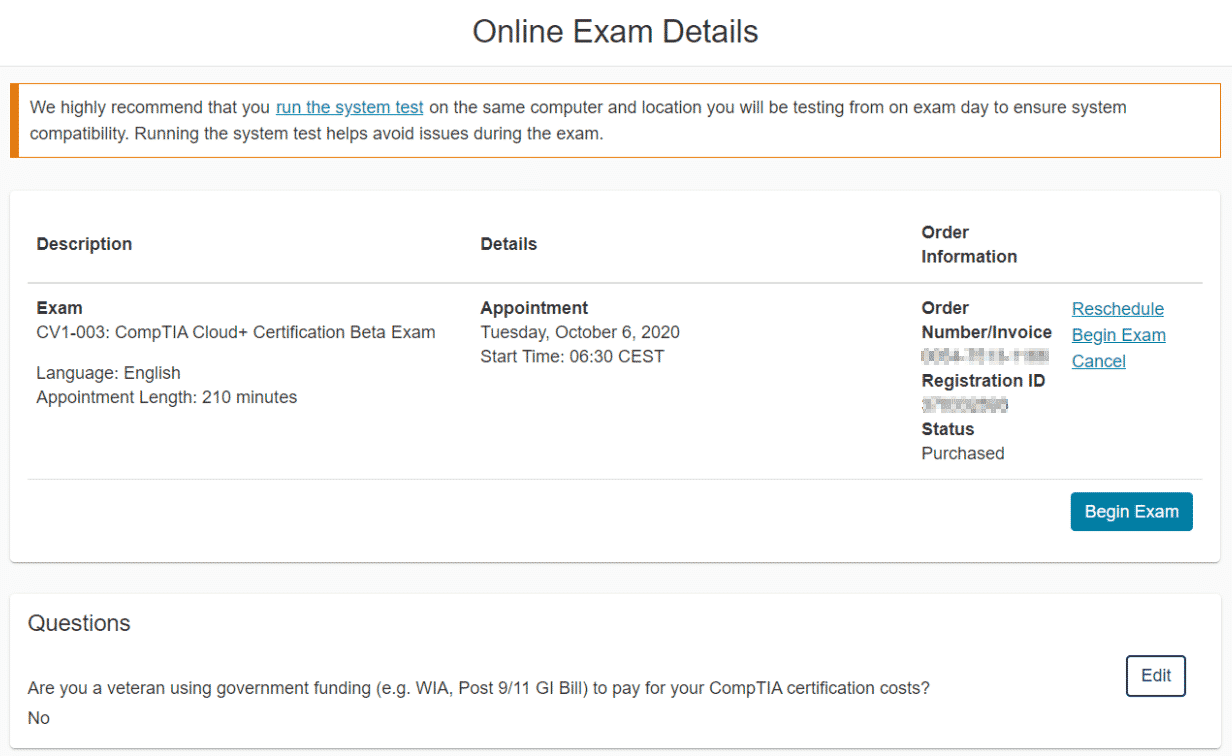The image details the "Online Exam Details" page. The header box, which is emphasized with an orange outline, is thicker on the left side compared to the top, bottom, and right sides. Within this box, there is a blue-highlighted note recommending that users run a system test on the same computer and at the same location they will use on the exam day to ensure compatibility and to avoid technical issues.

Below this header, on a gray background, there is a white box containing key details of the exam. The section titled "Description" states that the exam language is English and the appointment length is 210 minutes. The appointment is scheduled for Tuesday, October 6, 2020, with a start time of 6:30 CEST. 

Further below, under "Order Information," you can find sections for order number, invoice, registration ID, and status (which is marked as "Purchased"), though these numbers are obscured.

Options to reschedule, begin the exam, or cancel are available and displayed in blue, underlined text, indicating they are clickable. A prominent blue button labeled "Begin Exam" is also present.

Lastly, there is a section with a question asking, "Are you a veteran using government funding to pay for your CompTIA certification costs?", with the provided answer marked as “No.”